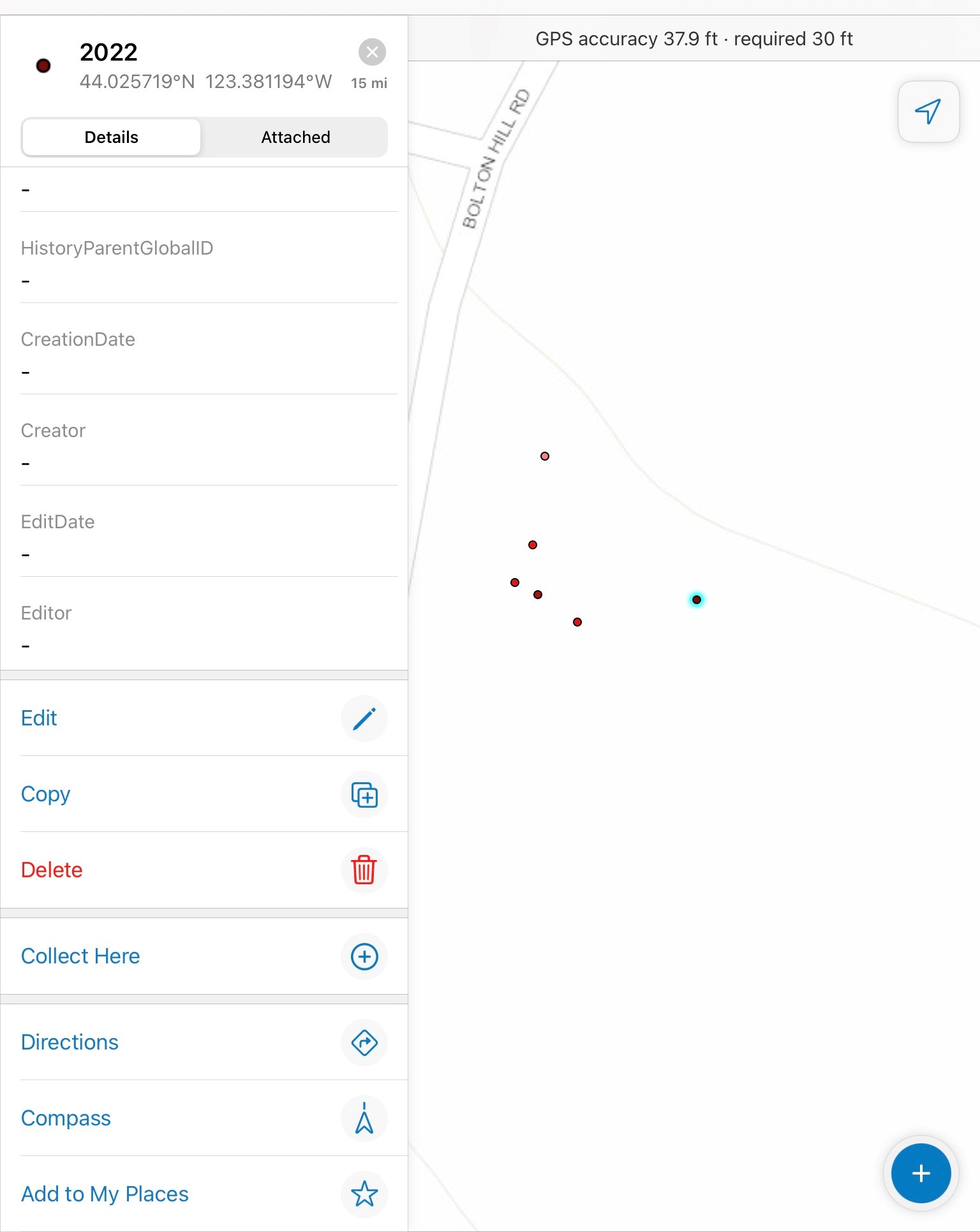A detailed and cleaned-up caption for the image could be:

"This image depicts a map locator application. At the top, the year "2022" is displayed alongside geographic coordinates "44.025719° N, 123.381194° W" and a distance indicator of '15 miles'. Below, there are two buttons labeled 'Details' and 'Attached'. A vertical menu on the left side of the screen features various options separated by dash marks: 'History', 'Parent', 'Global ID', 'Creation Date', 'Creator', 'Edit Date', and 'Editor'. Additional options within the menu are color-coded: 'Edit' (blue with a pen icon), 'Copy' (blue with a plus box icon on the right), 'Delete' (red with a trash can icon), 'Collect Here' (blue with a plus sign in a circle), 'Directions' (blue with a turn arrow), 'Compass' (blue with a navigation arrow), and 'Add to My Places' (blue with a star icon).

To the right, a map area is displayed, largely blank. Streets are identified in the upper left-hand corner, including 'Bolton Hill Road'. In the upper right-hand corner, a navigation arrow in a curved square icon is visible. The bottom of the map indicates GPS accuracy of '37.9 feet' with a required accuracy of '30 feet'. Five or six waypoints, marked as red dots, are scattered across the map. One of these waypoints is highlighted in blue. At the bottom right of the map, there is a white plus sign inside a blue circle."